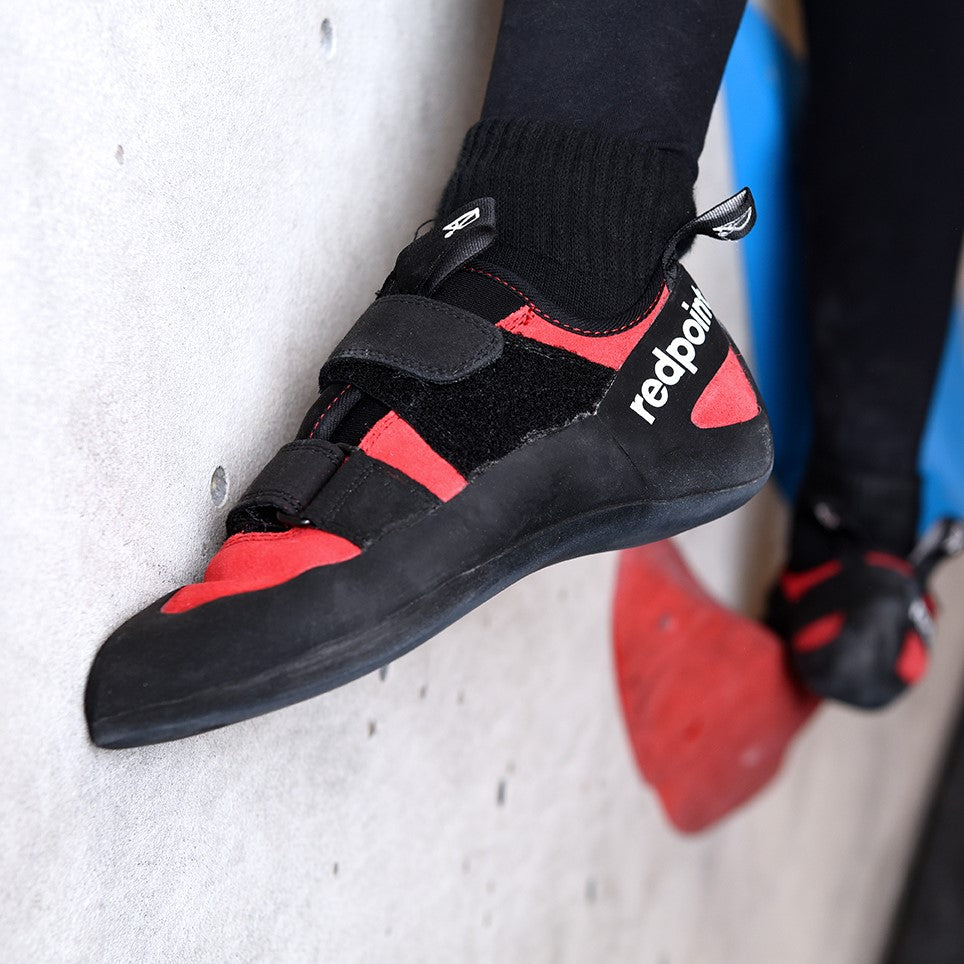The photograph depicts a close-up view of a rock climber's feet as they navigate a climbing wall. The focus is on the climbing shoes, which are predominately black with pinkish-red accents and feature bold white lettering that spells "red point" on the heels. One shoe is firmly planted on a protruding red hold on the white wall, while the other hovers in mid-air. The climber is wearing black socks and black leggings. The image also captures several openings in the climbing wall and a blurred blue element in the background, adding to the gym-like environment. The shoes have a unique strapping system with velvet straps zipped in the front for securing them tightly.